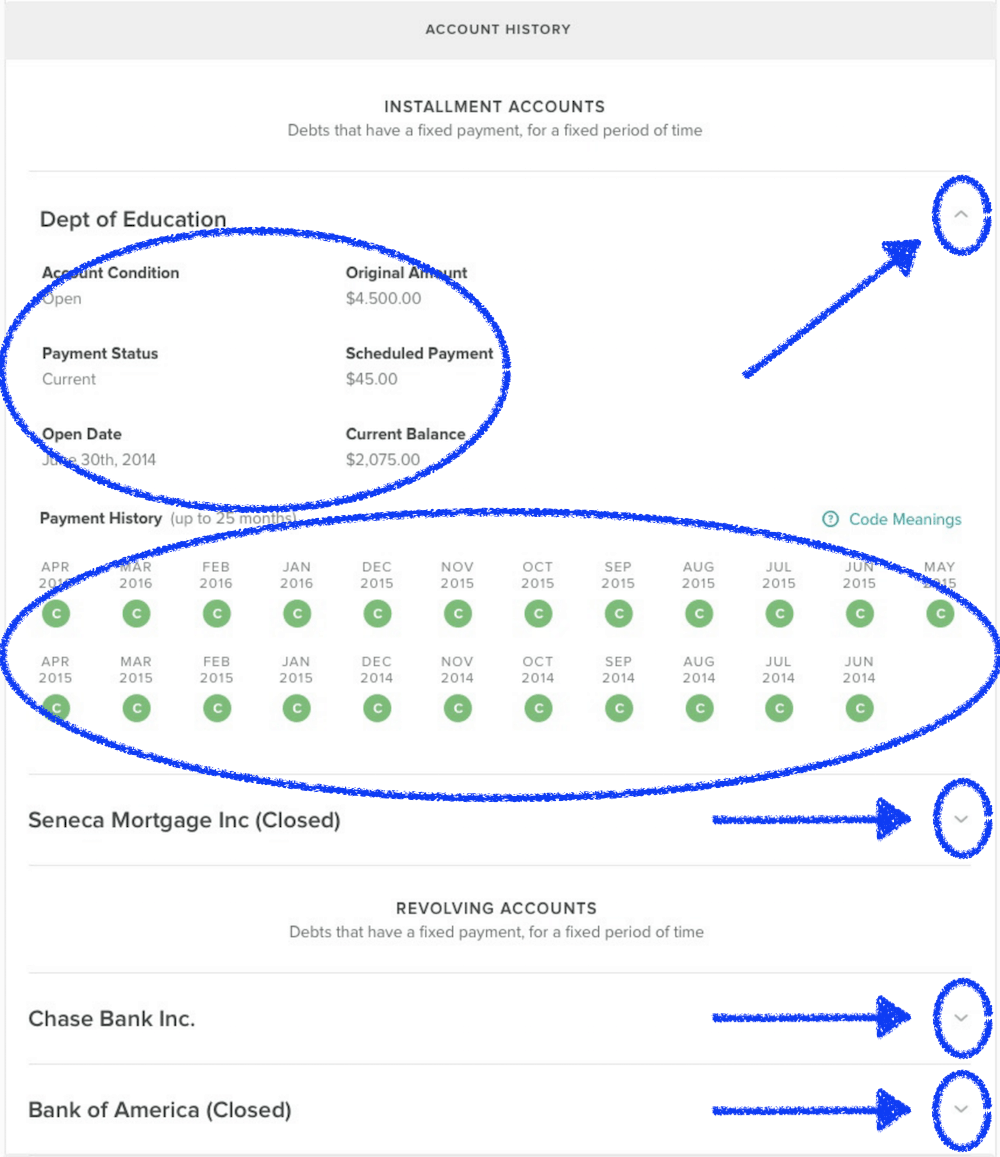This image is a detailed online account summary page. The page is in a portrait, rectangular format, approximately 30% taller than it is wide. 

**Header Section:**
- The header spans the entire width of the image with a light gray background. 
- In the center of the header, in small dark gray all-caps font, it reads "ACCOUNT HISTORY."

**Main Body:**
- Below the header, the background turns white and is bordered by thin gray lines on the left, bottom, and right sides.
- At the top center of the white field, the title "INSTALLMENT ACCOUNTS" is displayed in dark gray all-caps font, larger than the header font.
- Below this title, center-justified, it reads "Debts that have a fixed payment, for a fixed period of time" in regular sentence case font.
- A long, thin gray underline runs from left to right beneath this description.

**Account Details:**
- In the top left corner of the main body, the text "DEPT of Education" is displayed in dark gray font, with the 'D' and 'E' in uppercase and the rest in lowercase, sans period after 'DEPT.'
- The account details are arranged in two columns, each containing three fields:
  - **Left Column:** 
    1. Account Condition (Bold) - Open
    2. Payment Status (Bold) - Current
    3. Open Date (Bold) - June 30, 2014
  - **Right Column:** 
    1. Original Amount (Bold) - $4,500.00
    2. Scheduled Payment (Bold) - $45.00
    3. Current Balance (Bold) - $2,075.00
- Surrounding these fields, a chalky medium blue oval encapsulates most but not all fields, leaving some corners cut off for a stylized effect.

**Upper Right Corner:**
- An upward-facing arrowhead, in very light gray, is encircled by a chalky medium blue egg-shaped form.
- This encapsulated arrowhead features a long line angling down at approximately 45 degrees towards the lower left.

**Payment History:**
- In the upper left of the middle section, it reads "PAYMENT HISTORY" in bold, followed by "UP TO 25 MONTHS" in parentheses, non-bold.
- This section features two rows of dates:
  - **Top Row:** Starts with APR2016 on the left, ending with MAY2015 on the right. Each date has a green circle with a white ‘C’ below it.
  - **Bottom Row:** Starts with APR2015 on the left, ending with JUN2014 on the right, containing one less date, leaving a blank spot beneath MAY2015.
- A long chalky medium blue oval encircles these dates, overlapping some lines but covering all the green circles.

**Additional Sections:**
- Below the payment history section, there are four rows:
  - **First Three Rows:**
    1. Seneca Mortgage, Inc. (CLOSED)
    2. Chase Bank, Inc.
    3. Bank of America (CLOSED)
  - Each of these rows features a downward-facing gray arrowhead circled with an egg-shaped blue form with a horizontal arrow pointing leftwards.
- **Text Between First and Second Rows:**
  - Center-justified bold all-caps text reads "REVOLVING ACCOUNTS."
  - Below it, "DEBTS THAT HAVE A FIXED PAYMENT, for a fixed period of time" is displayed in regular font.